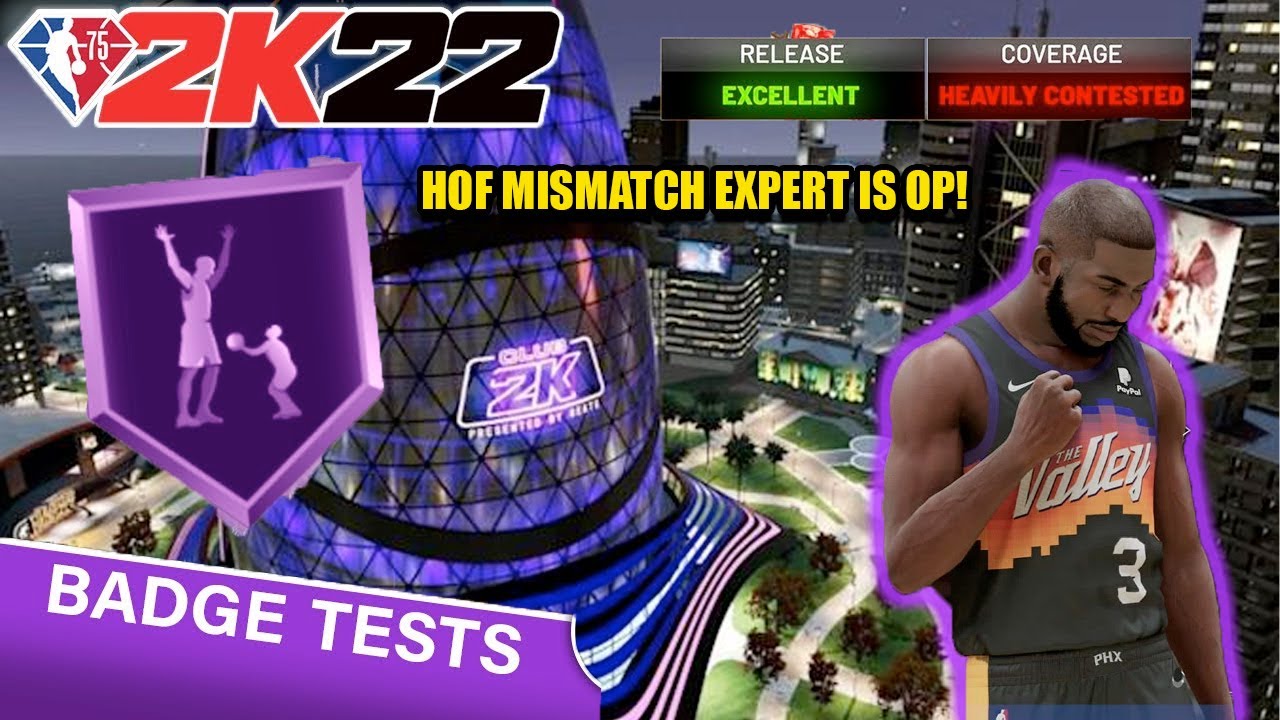The image shows a vibrant advertisement banner with a complex design set against a dark background, accentuated by an array of colors and details. At the top part, resembling a night sky with a deep bluish hue, the upper left-hand corner prominently features the NBA logo. This logo is diamond-shaped, split into blue and red halves with a white outline, showcasing the iconic silhouette of a basketball player—probably Michael Jordan—holding a white basketball. 

Beneath the logo, the text "2K" appears in bold red with a white outline, followed by "22" in black, also outlined in white. Below this, the area transitions to black, featuring the text "HOF Mismatch Expert" in vibrant yellow, outlined in black, and emphasized with an exclamation point.

In the bottom left corner, a purple section contains the words "batch test" in crisp white letters. The right side of the image reveals a futuristic building labeled "Club 2K," constructed predominantly of glass and illuminated with purple, white, and blue lights. The ground below is green, interspersed with green and red trees, and beige walkways meander through the scene.

To the right, additional buildings stand tall with dark exteriors but bright, colorful lights. Some of these buildings display advertisements in various colors such as blue, white, and brownish hues, although the specific content of these ads is indiscernible.

On the right-hand side, a striking image of a man with a dark complexion is visible. He wears a blue jersey marked with the number three and the word "The Valley." The man, who has a black beard, raises his fist and sports a confident smirk. In the final touch, outlines of animated armatures frame the right corner of the image, adding to the dynamic and engaging composition.